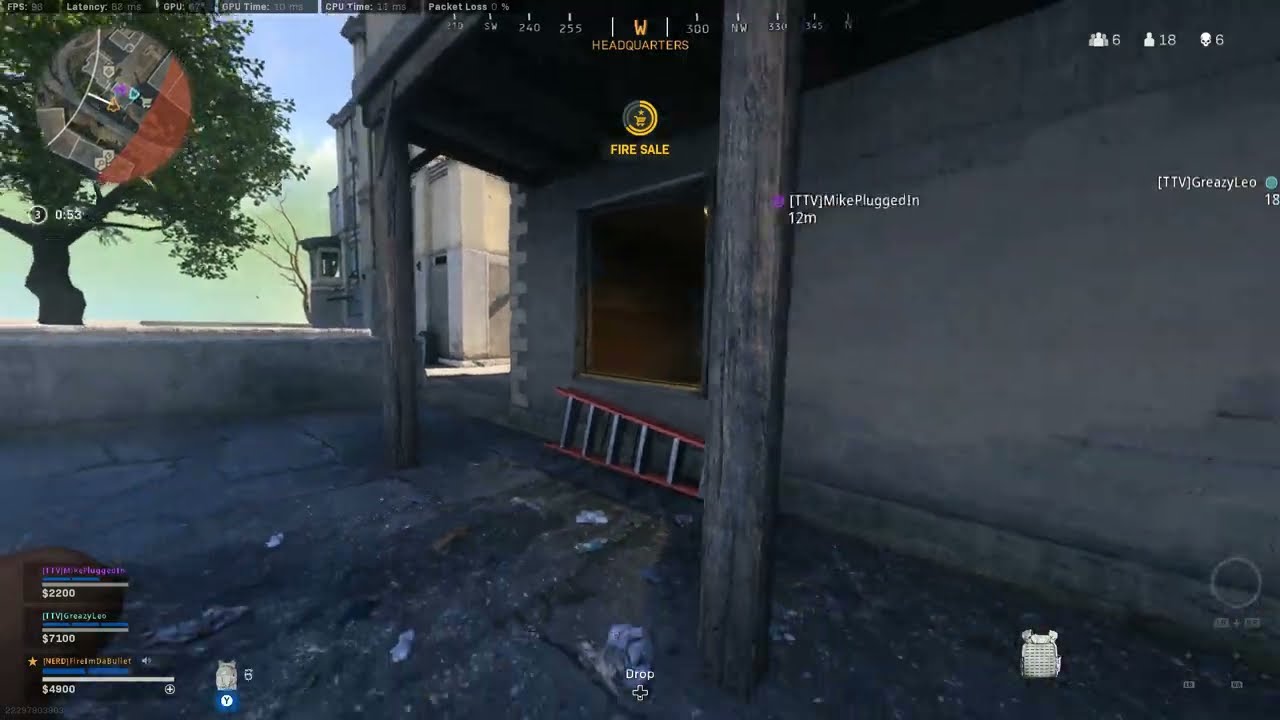The image is a highly detailed color still shot from a first-person shooter video game, showcasing a rustic two-story building with a dilapidated stucco facade in gray. The second-floor balcony, supported by large gray wood beams, draws attention, and a red ladder with silver steps leans against the building beneath a window. Next to the main structure, there's another gray building in the distance, and to the left, a large green oak tree stands out against the blue sky. 

In the gaming interface, "FIRE SAIL" is prominently displayed in yellow near the top center, with "Headquarters" visible above it. The top right corner indicates six players are participating, with scores and usernames such as "Mike Plugin 12M" displayed in white text. The bottom left corner features bar graph scores and price tags reading $2,200, $7,100, and $4,900 in white text, likely representing players' in-game resources or points. The setting exudes a photographic illustration style, blending the rustic environment with the immersive, interactive elements of the video game.